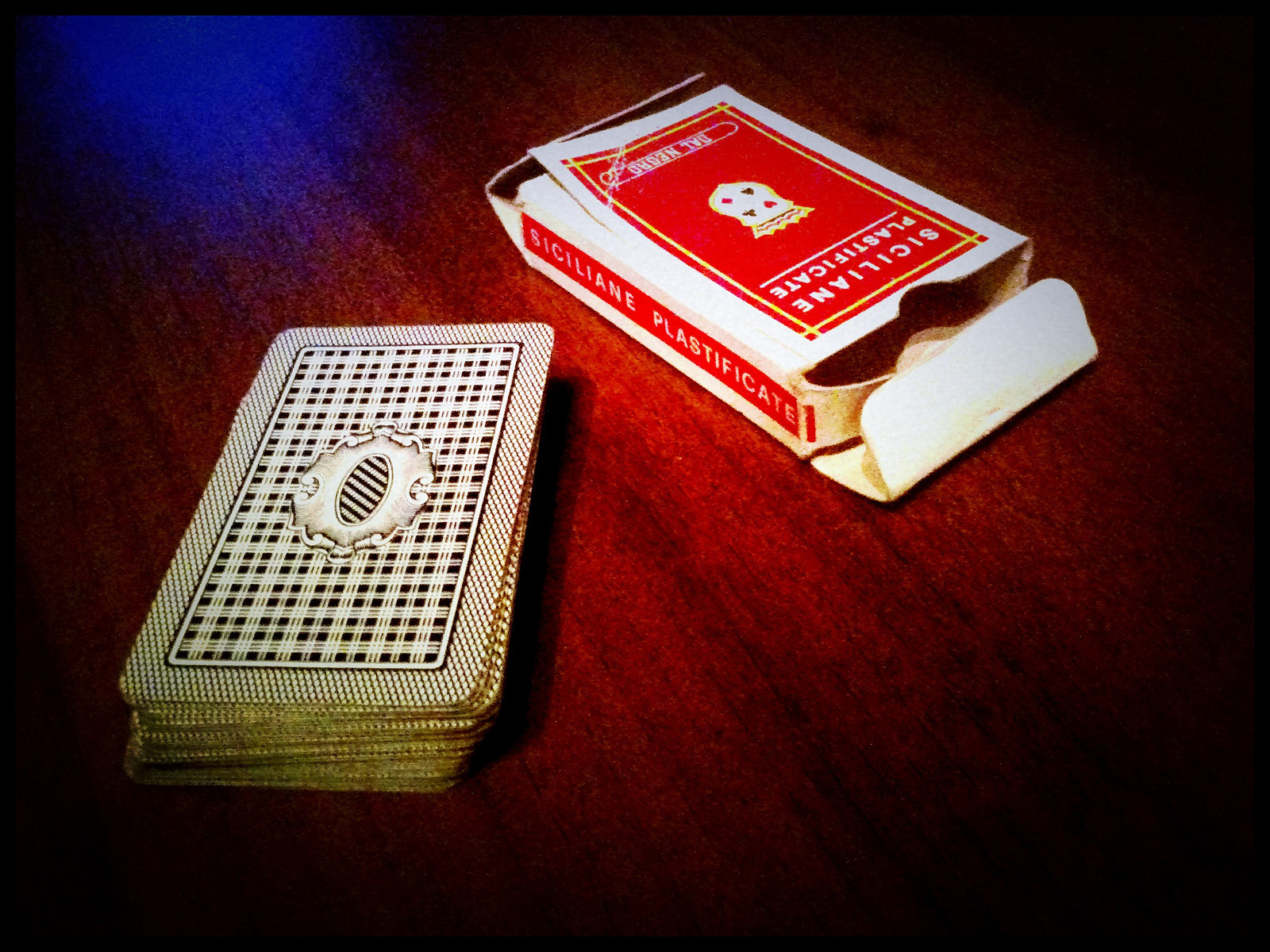On a rich, mahogany table rests a neatly stacked deck of intricately designed cards. These cards, removed from their box, are positioned on the left side at a slight angle. Each card features an elaborate black and white pattern, with a small checked border encompassing the card's edges. Inside this border lies a rectangular area adorned with a black and white plaid pattern. At the very center of the card, a silver medallion with scalloped edges draws the eye. Within this medallion, an oval with striking black and white stripes completes the design.

Adjacent to the cards is the box that housed them. The box is predominantly white, with a large red rectangle on the top and a narrow red stripe on the side. The side stripe is inscribed with the word "SICILIANE" in bold letters, followed by "plasticate". The top of the box also reads "plasticate" within the red rectangle and features a shield emblazoned with hearts, diamonds, clubs, and spades. The box shows signs of wear and tear, with openings at both ends and the bottom left corner beginning to come apart, adding a hint of rustic charm to the setting.